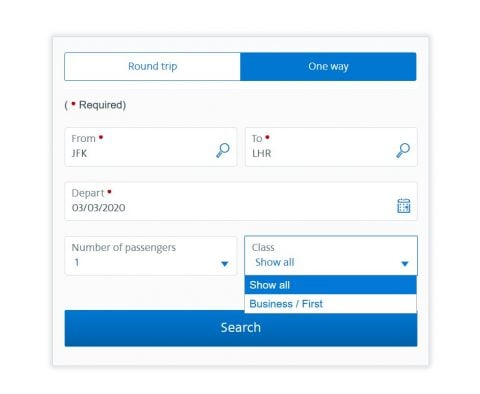This image showcases a segment of a travel booking webpage, specifically designed for planning trips. The central focus is a minimalist white box with a subtle gray trim. At the top of this box, users are presented with two options: "Round Trip" and "One Way." These options are displayed in blue text within smaller, softly highlighted rectangular buttons. The "One Way" option stands out as it is selected, thus its background is blue and the text is white.

Directly below these options, the word "Required" appears, enclosed in parentheses and marked with an asterisk to indicate a mandatory field. The subsequent fields display journey details filled out by the user: the departure is set from JFK (John F. Kennedy International Airport) to LHR (London Heathrow Airport). The departure date is listed as 03/03/2020, and the number of passengers is specified as one. There is also a "Class" dropdown menu currently set to "Show All."

Beneath these details, a prominent blue search button invites users to commence their search for available flights. The overall layout of the box is straightforward and intuitive, designed to facilitate easy travel booking. Should the user click the search button, they would be presented with various flight options for the specified one-way trip from JFK to LHR. If the "Round Trip" option were selected instead, additional fields for return flight details would appear. This clean and user-friendly interface is typical of online travel booking platforms.